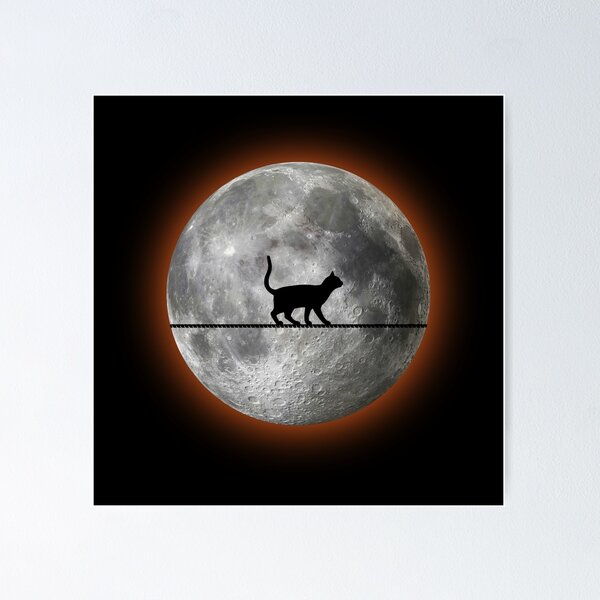The image depicts a striking, digitally created scene of a black, silhouetted cat walking on a tightrope in front of a detailed moon. The moon is gray with dark spots, white cracks, and a few visible craters, particularly on its lower portion. Encircling the moon is a vivid red or orange ring, giving the scene an eclipse-like appearance. The entire background of the image is a deep black, and the square image appears to be hanging on a white wall. The cat is positioned centrally on the tightrope, facing to the right, with its tail raised. The elements combine to create a visually captivating, surreal composition without any accompanying text.